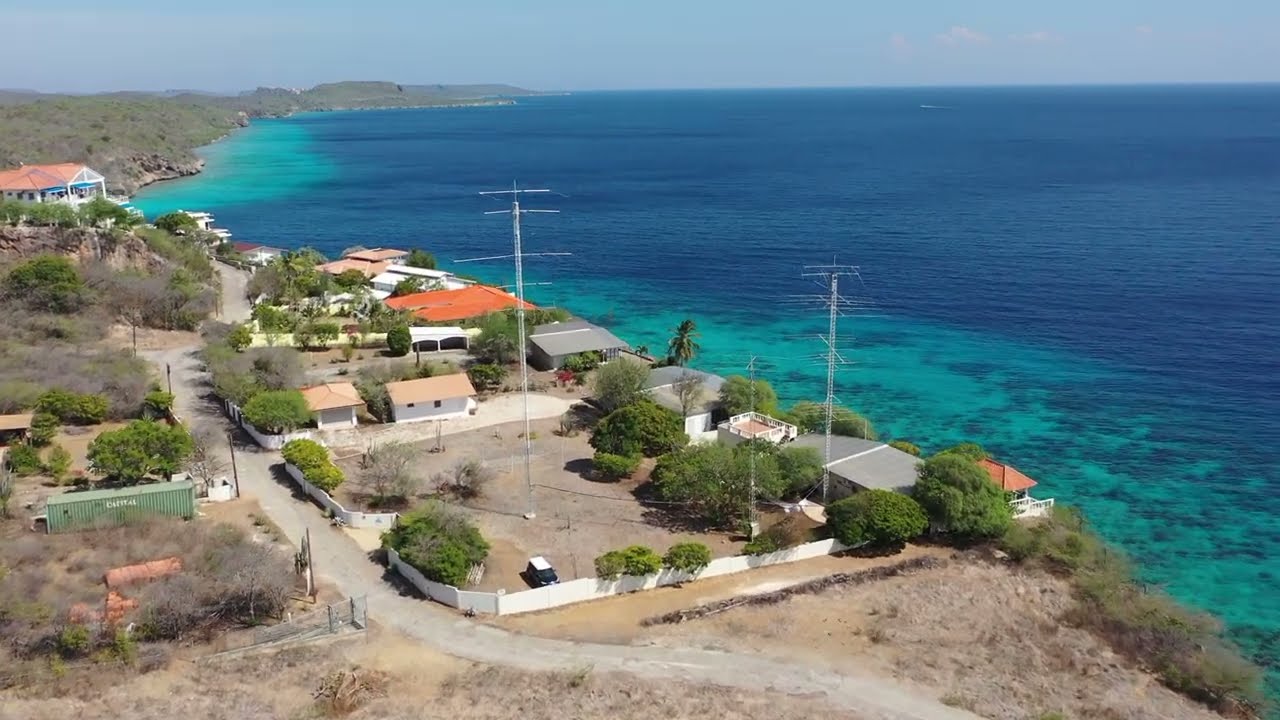The image showcases a serene coastal scenery featuring a stretch of one-story houses situated along a dirt road that winds alongside a beautiful, inviting body of water. The water exhibits a gradient of colors, starting with light turquoise near the shore and transitioning to dark blue as it extends into the distance. This large body of water, taking up approximately 60% of the picture, suggests an ocean or possibly a lake, with no visible boats.

The terrain around the houses includes sandy backyards, scattered shrubbery, and white fencing that encloses many of the properties. Notable details include a cargo container located off to the left of the roadway, and a small peninsula of land jutting into the water in the upper left-hand corner of the image. The overall scene is very flat, with a clear sky providing a peaceful backdrop. The brown dirt road not only allows for vehicle access but adds to the rustic charm of the area, making it a picturesque and inviting location ideal for swimming, boating, or kayaking.